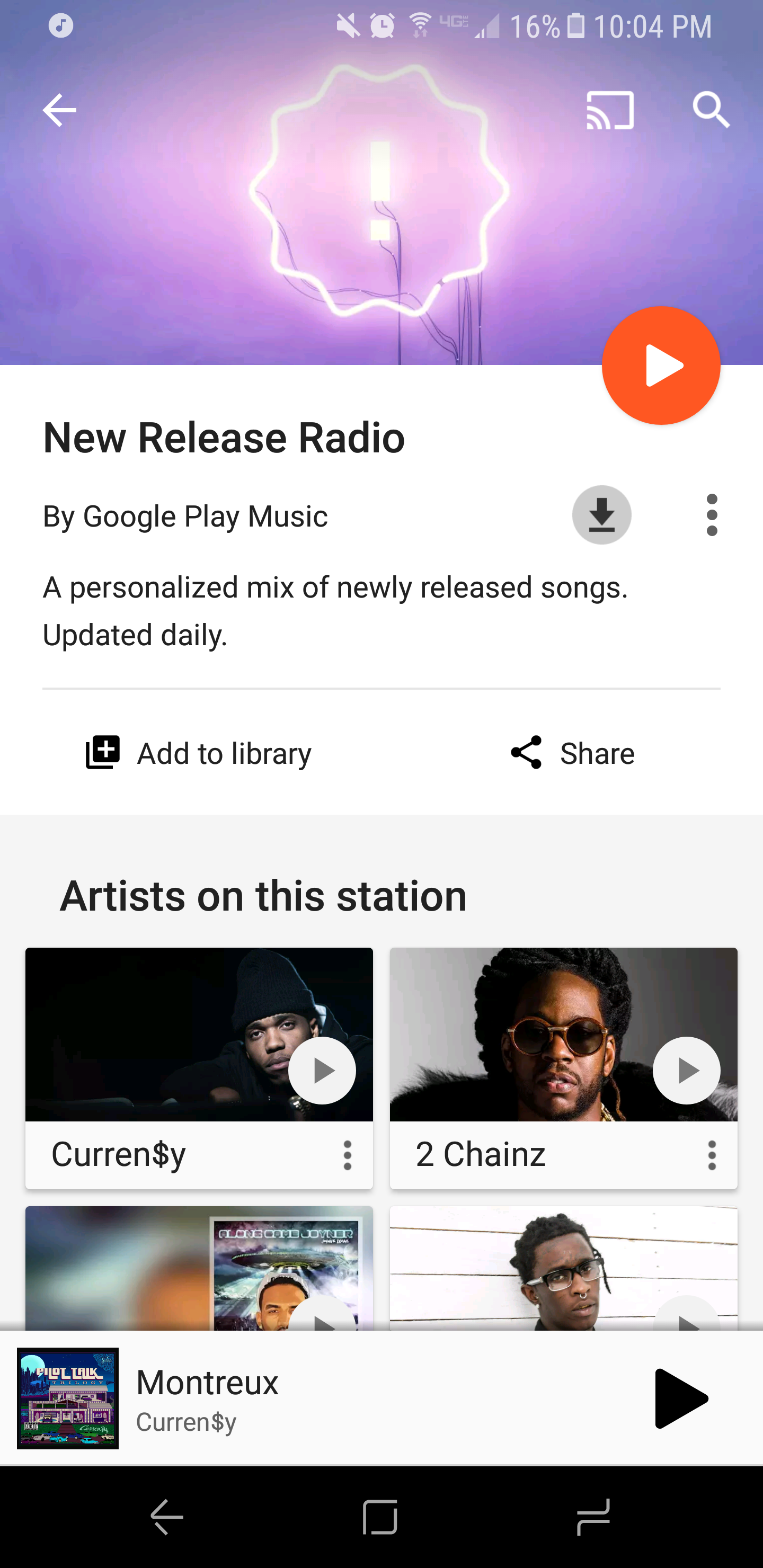The screenshot, taken on a mobile device at 10:04 PM, displays various indicators: a 16% battery level with no charging activity, an alarm clock icon, and the phone's sound set to silent. The top of the screenshot features a vibrant purple image with a neon exclamation mark encircled by a ten-sided star pattern. Below this, there's a white box highlighting "New Release Radio" by Google Play Music, described as a personalized mix of newly released songs, updated daily. A prominent red button with a white play triangle occupies the center, accompanied by options to "Add to library" and "Share." Further down, the section labeled "Artists on the Station" lists artists, starting with Curren$y, a young black man wearing a black beanie in a dimly lit room. The next artist is 2 Chainz, depicted as a black man with an afro and sunglasses. The currently playing artist is Curren$y, with the song titled "M-O-N-T-R-E-U-X."